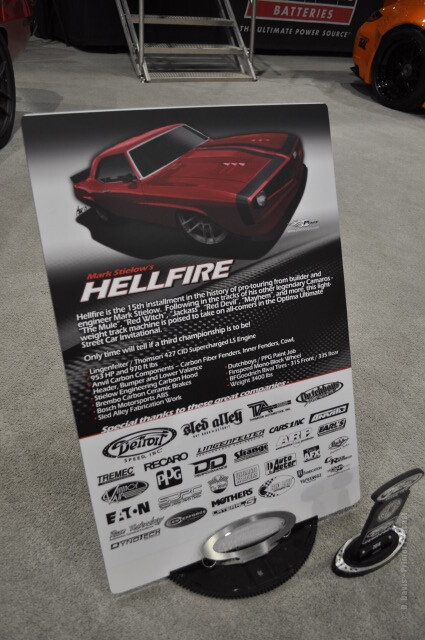This photograph captures a display setup on the floor of a garage. In the upper right corner of the image, a sports car with an orange exterior and a black wheel is partially visible, hinting at the setting's automotive theme. The focal point of the photograph is a small pamphlet held up by a plastic pedestal. The pamphlet features a striking image of a red 1969 Camaro with a black stripe, labeled with the name "Hellfire"—one of the legendary cars designed by builder and engineer Mark Stieglow. The text on the pamphlet highlights that "Hellfire" is the 15th installment in Stieglow's pro-touring history, following iconic builds like the Mule, Red Witch, Jackass, Red Devil, and Mayhem. This lightweight track machine is geared up for the Optima Ultimate Street Car Invitational, boasting a supercharged LS engine with 953 horsepower and 970 foot-pounds of torque. The bottom section of the pamphlet displays various sponsor logos, including Detroit Speed Inc., Tremec, and Eaton. Adjacent to the pamphlet stands an award, further emphasizing Hellfire's prominence in the competitive street car scene.